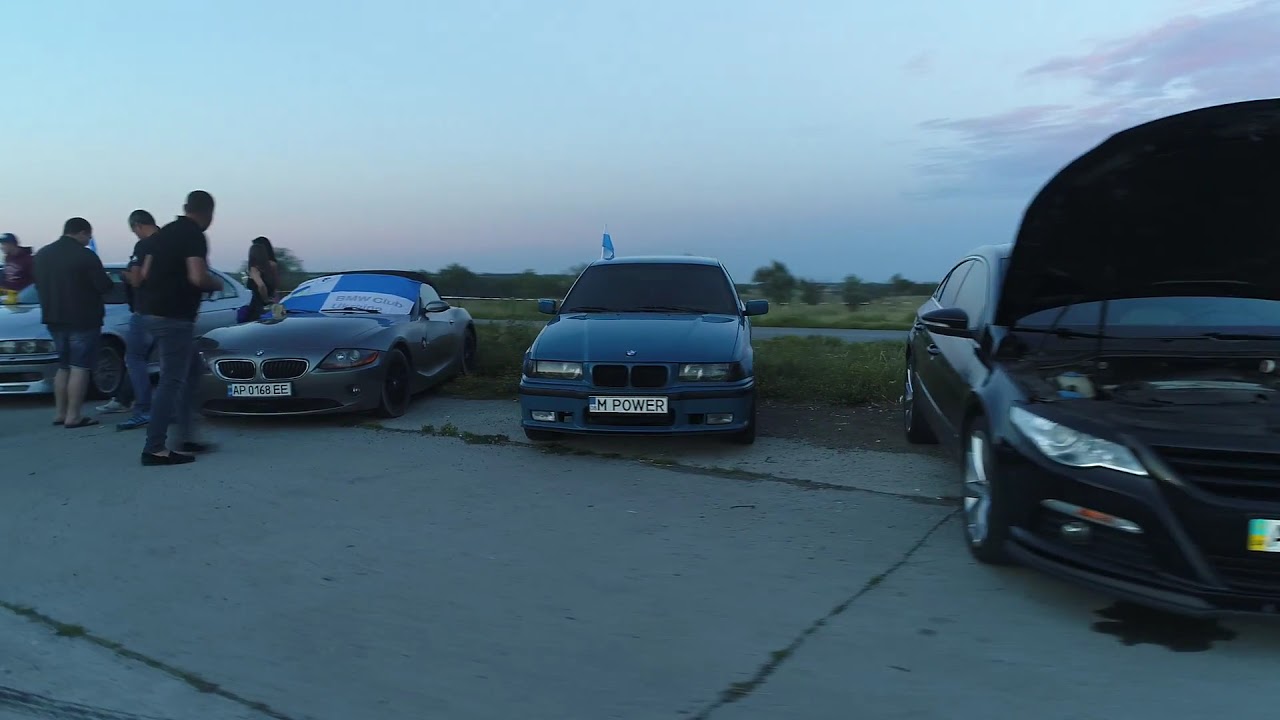In the image, there are four cars lined up side by side on a concrete surface with some grass and a distant road behind them. The sky above shows a gradient of light blue to pink, suggesting a sunset. The car on the far right is black with its hood open, revealing the engine, and has a license plate with a blue and yellow design on the right edge. In the center is a light blue BMW with squarish headlights and a license plate that reads "M Power" in black text on a white background. This car also has a flag attached to the left side of its roof. To the left of the blue BMW is a silver car with a blue and white checkered windshield cover and a white license plate that has "AP 016AEE" in uppercase letters. Further to the left is a white car, also a BMW, with a sports car design. In front of the two leftmost cars stands a group of five light-skinned people wearing dark-colored tops. The group includes one woman on the right and four men, two of whom are in jean trousers and one in jean shorts. The scene suggests a car show, with the audience admiring the vehicles on display.